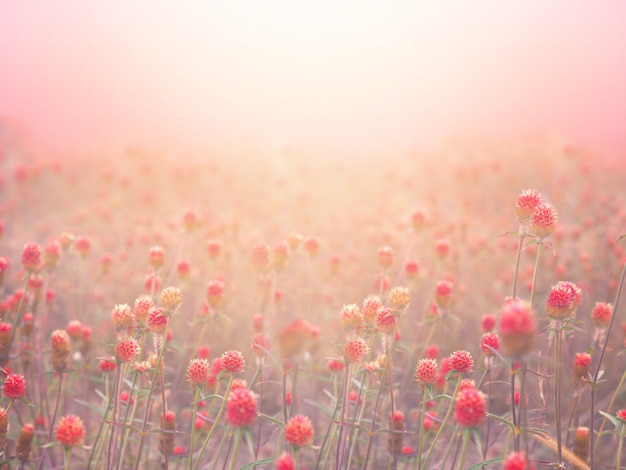This image, which appears to be a detailed photograph or a highly realistic painting, depicts a vast field filled with countless flowers. Each flower features a distinctive bulbous red or pink bloom atop tall, slender green stalks. The foreground flowers are rendered in sharp focus, showcasing their intricate, spiky clusters of micro-petals, but they gradually fade into a soft blur as the field stretches into the distance, giving an impression of a mist or light fog permeating the area. The overall composition is bathed in a bright, diffused light that seems to emanate from an intense sun positioned at the upper center of the image. This sunlight not only casts a golden hue over the scene but also partially washes out the upper portion, blending into a vague blue sky with hints of pink, enhancing the ethereal and dreamlike quality of the landscape.